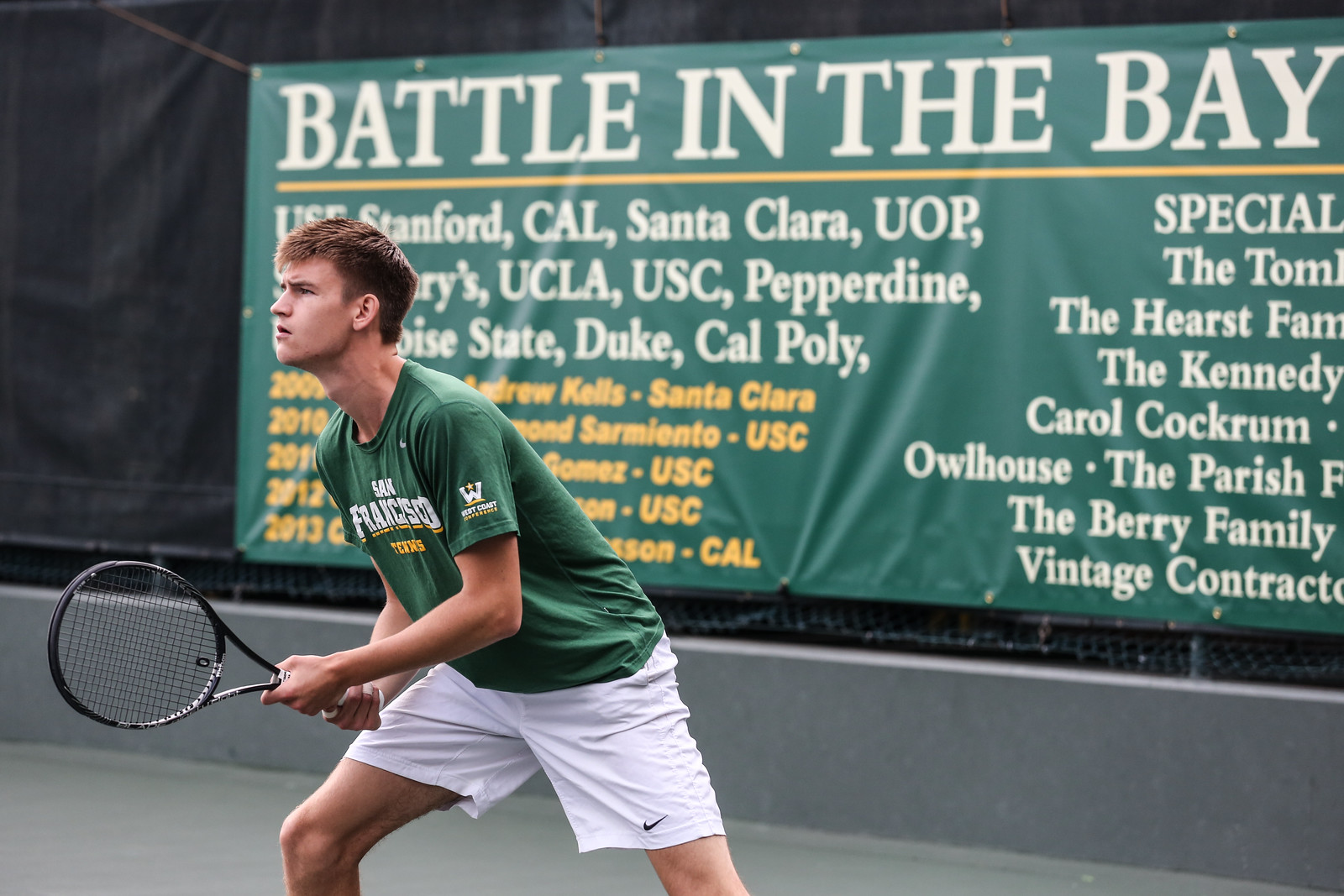The image captures a young man, a tennis player, in a green t-shirt uniform that reads "San Francisco" with "tennis" written beneath in yellow text, and "West Coast Conference" on the sleeve. He is gripping a tennis racket with both hands in front of his body, poised in a ready stance, possibly preparing to return a serve or intensely focused on the other side of the court. He is also wearing white Nike shorts. The tennis court features a gray cement wall about two feet tall with a net or fence above it. A green tarpaulin banner in the background displays "Battle in the Bay" at the top, along with names of participating schools and sponsors, including USB Stanford, Cal, Santa Clara, UOP, UCLA, USC, Pepperdine, State schools, Duke, Cal Poly, and various family and business sponsors, all in white and yellow lettering.